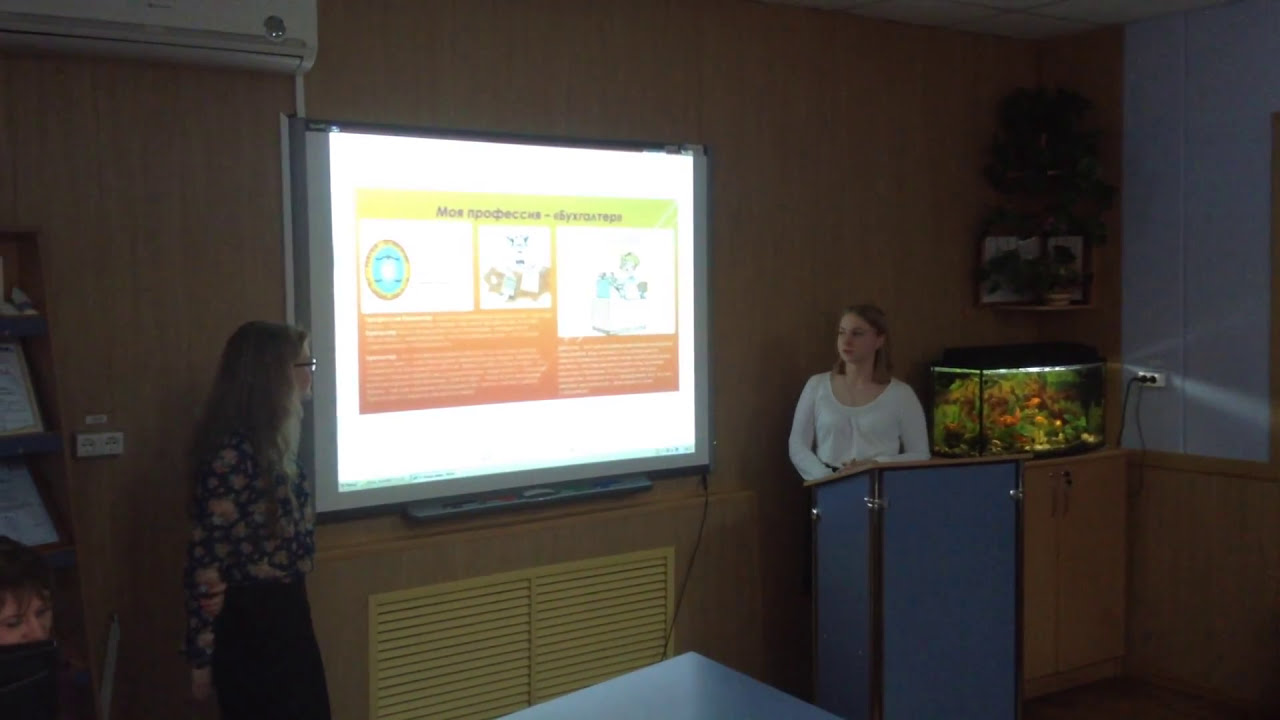The photograph depicts a classroom setting featuring two young women engaged in what appears to be a PowerPoint presentation. The room has a distinct brown wood-paneled wall behind an illuminated projector screen showing a slide in a non-English language, with graphic elements and a yellow and orange design. Standing at a blue-colored podium with a wooden top on the right side of the room is a woman with shoulder-length, light brown hair, wearing a white long-sleeve shirt. Next to her, on a stand, is an aquarium plugged into a nearby socket, with a shelf above it holding a picture and a plant. On the left side of the projector screen, another woman with long, wavy brown hair and glasses wears a floral long-sleeve blouse and black pants or skirt. She is facing the screen, adding to the scene's sense of interaction and focus.